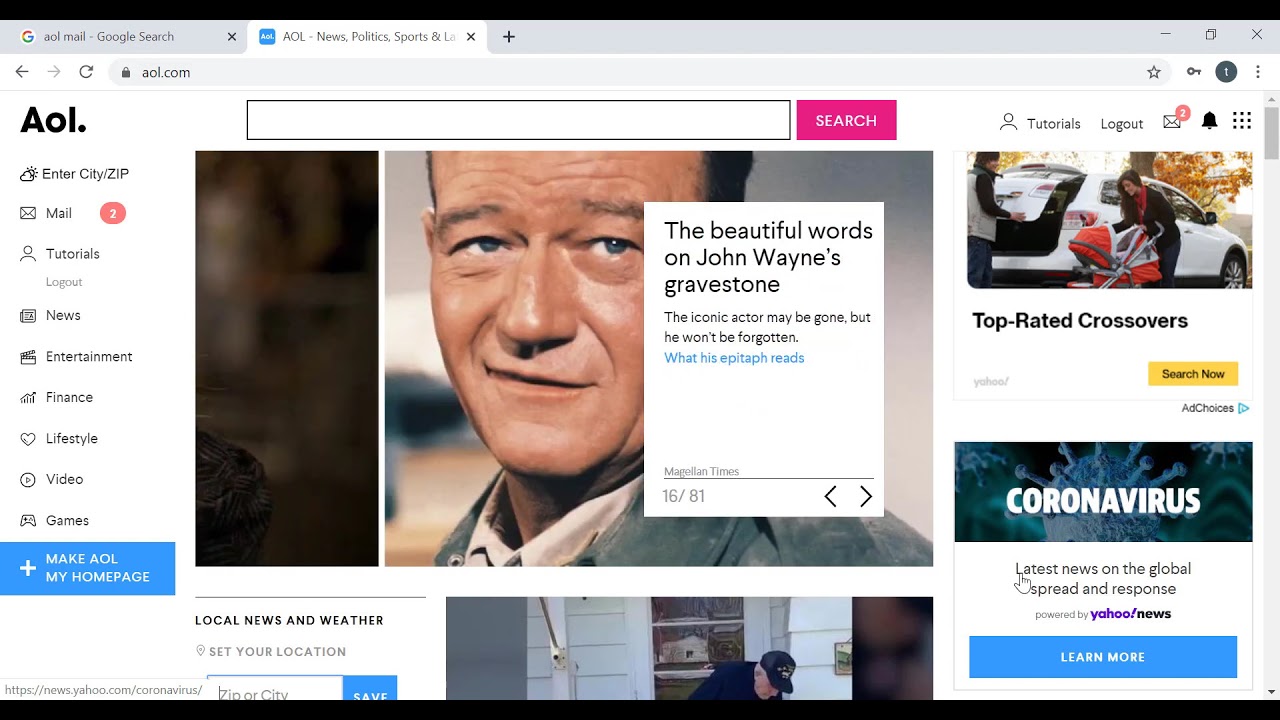The image displays the AOL homepage as viewed on a Microsoft Edge browser. The interface prominently features a serene white background with a search bar positioned at the top. On the left side of the screen, a section appears that seems to highlight a quote from John Wayne's gravestone. The page includes a variety of news content, with a sidebar dedicated to weather alerts and top-rated crossovers. Additionally, there are multiple news articles visible, providing a comprehensive snapshot of current events. Another tab is seen open in the Microsoft Edge browser, but the content of that tab is not fully legible.